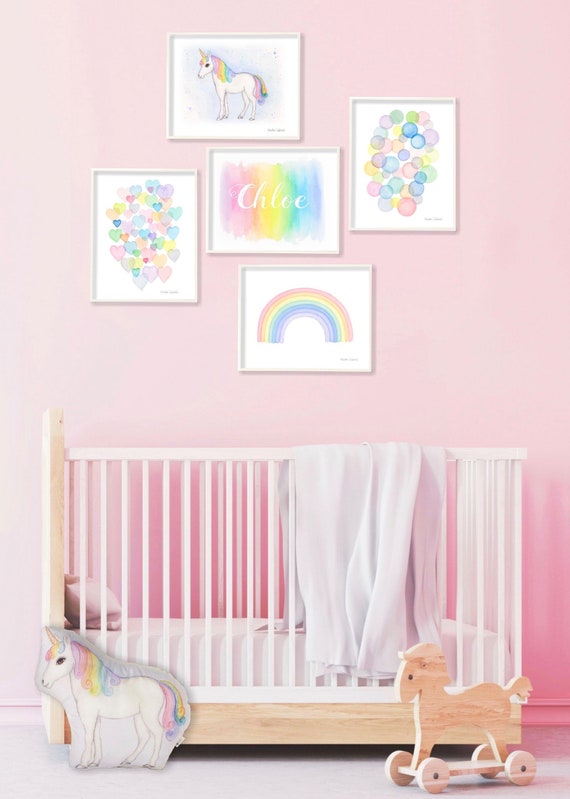The photograph captures a baby girl's nursery adorned in soft, light shades of pink. The back wall of the room is painted with a gentle pink hue and is embellished with five framed images, all in a harmonious pastel rainbow theme. The central image showcases the name "Chloe" written artistically in white script against a rainbow backdrop. Above it is a whimsical picture of a unicorn with a vibrant, rainbow-colored mane. To the left of Chloe’s name image is a frame filled with multicolored hearts, and to the right, a frame features an array of multicolored bubbles. Completing the set, at the bottom, there is a charming rainbow painting.

Below this gallery of artwork, a white and wood baby crib sits elegantly. The crib, featuring white slats and a wooden frame, is draped with a grayish-white blanket over one side. In the foreground of the picture, a wooden horse toy with wheels is placed prominently, accompanied by a colorful unicorn picture rested against the crib. The entire ensemble suggests a cozy, thoughtfully designed nursery with a playful yet soothing atmosphere, perfect for a little girl named Chloe.